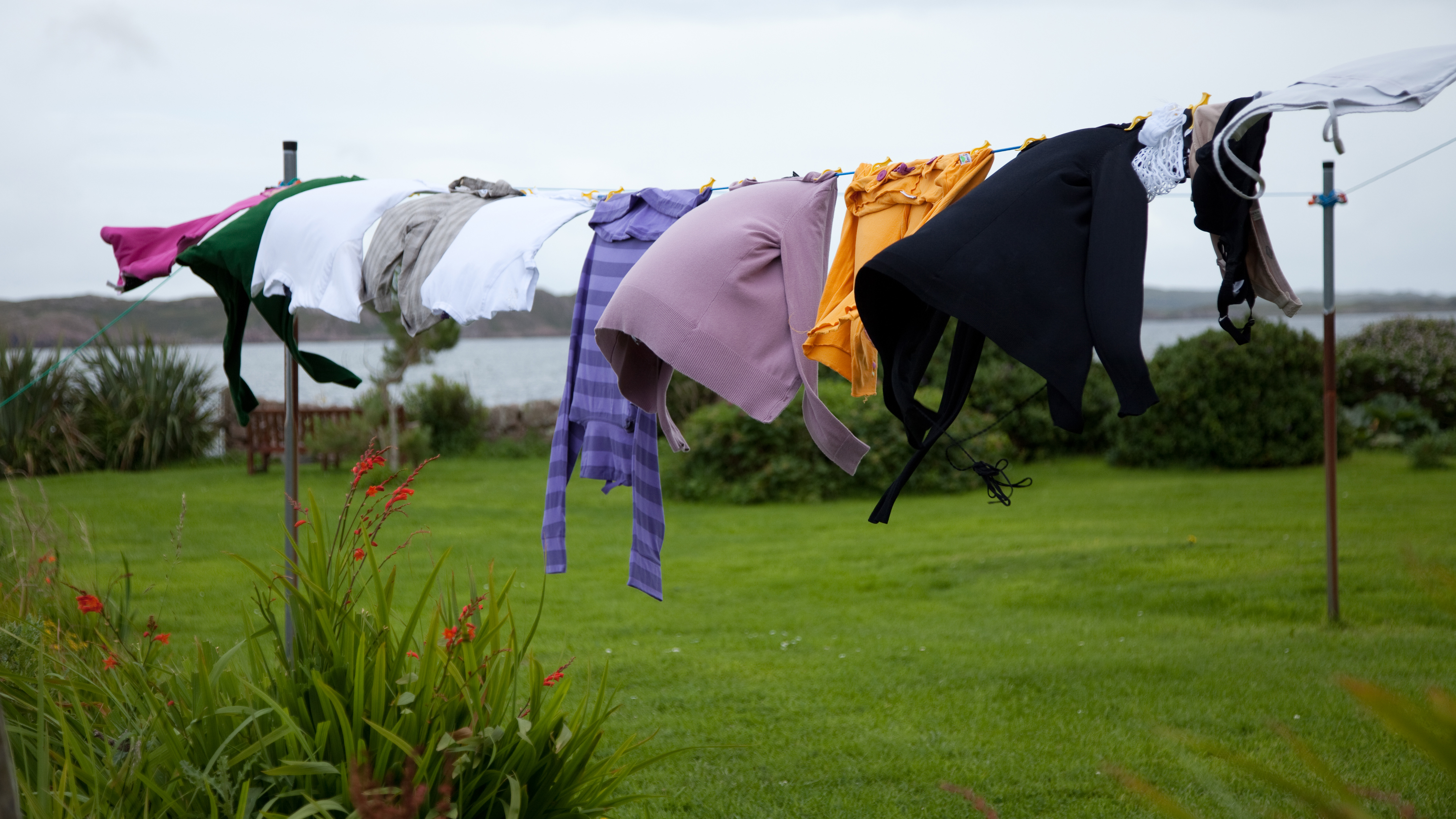The image captures a vivid and dynamic scene of a backyard clothesline set against a picturesque landscape. The primary focus is on a simple, rustic clothesline, held up by two rust-colored metal poles, with a white string stretched between them. Various pieces of clothing, including a light purple long-sleeve shirt, a pink sweatshirt, a black jacket, green sweaters, and white shirts, are clipped to the line with clothespins. The clothes billow to the left in the wind, giving a sense of movement.

Beneath the clothesline, the yard is a lush expanse of green grass. In the immediate foreground on the lower left side, tall, spear-like plants with striking red flowers punctuate the lawn. Just beyond the green expanse, there is a cluster of bushes and a quaint red wooden bench situated to the left.

Further into the background, the scene opens up to reveal a serene body of water, possibly an inlet bay or a wide river. Across the water, a range of hills or mountains rises majestically, providing a natural border under a muted, grayish-white sky. The combination of these elements— the vibrant lawn, the gently swaying clothes, and the dramatic natural backdrop—creates an atmosphere that is both tranquil and alive with the subtle rhythms of nature.